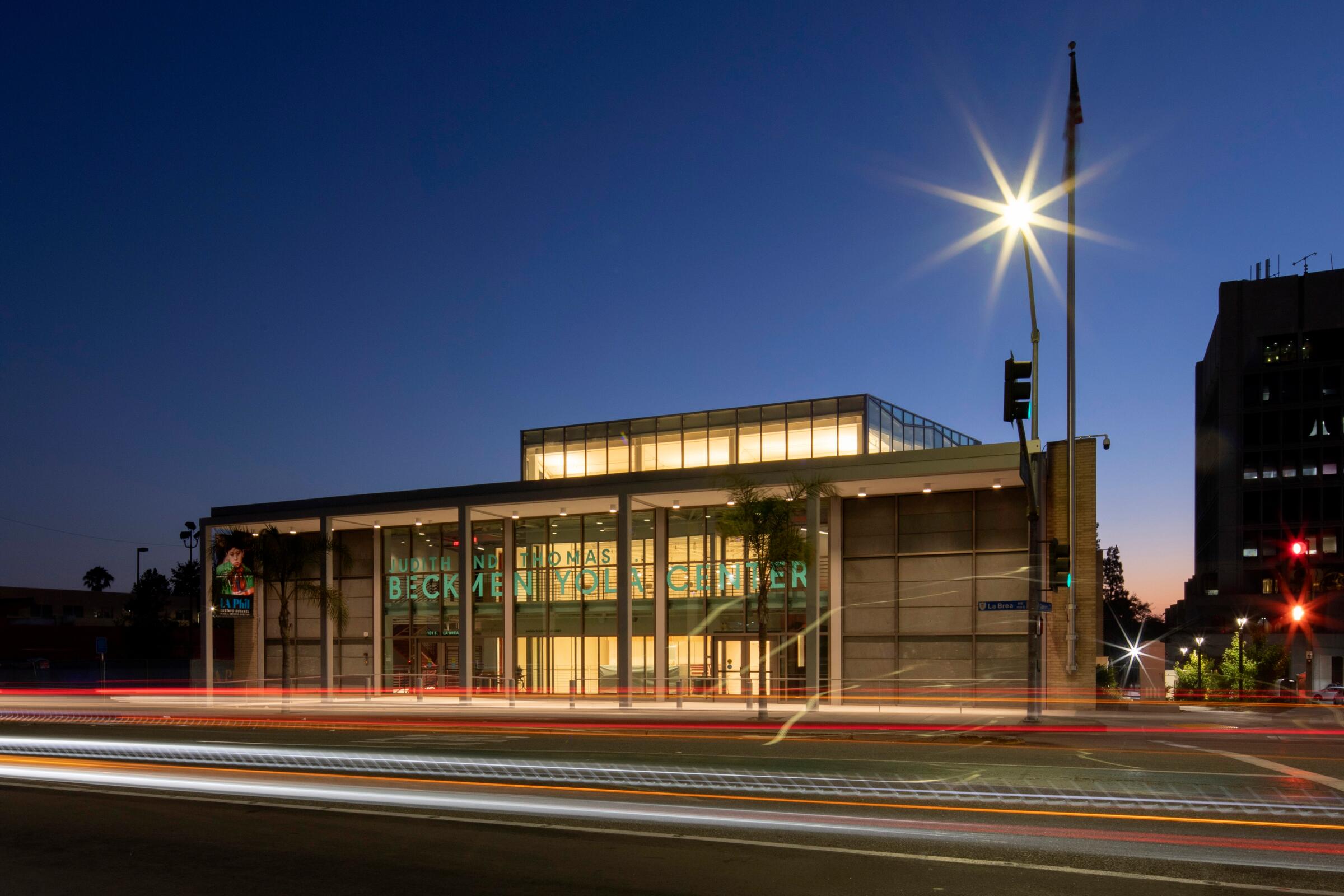This nighttime photograph captures a well-lit urban scene, prominently featuring the Judith and Thomas Beckman Yola Center. The building, situated at the corner of a bustling street, stands out with its glass-walled facade, including a second-story glass portion that only covers part of the structure. The green writing on the glass front is distinctly visible. Flanked by stoplights on both corners, the traffic signals add vibrant red and green hues to the image. Trails of headlights and taillights from passing cars streak across the foreground, a testament to the long exposure of the shot. An American flag on a flagpole is also noticeable on the right-hand side of the frame, illuminated by a streetlight. Off to the far right, a taller, mostly dark building with a few lit windows looms in the background, adding depth to the bustling nighttime city scene.